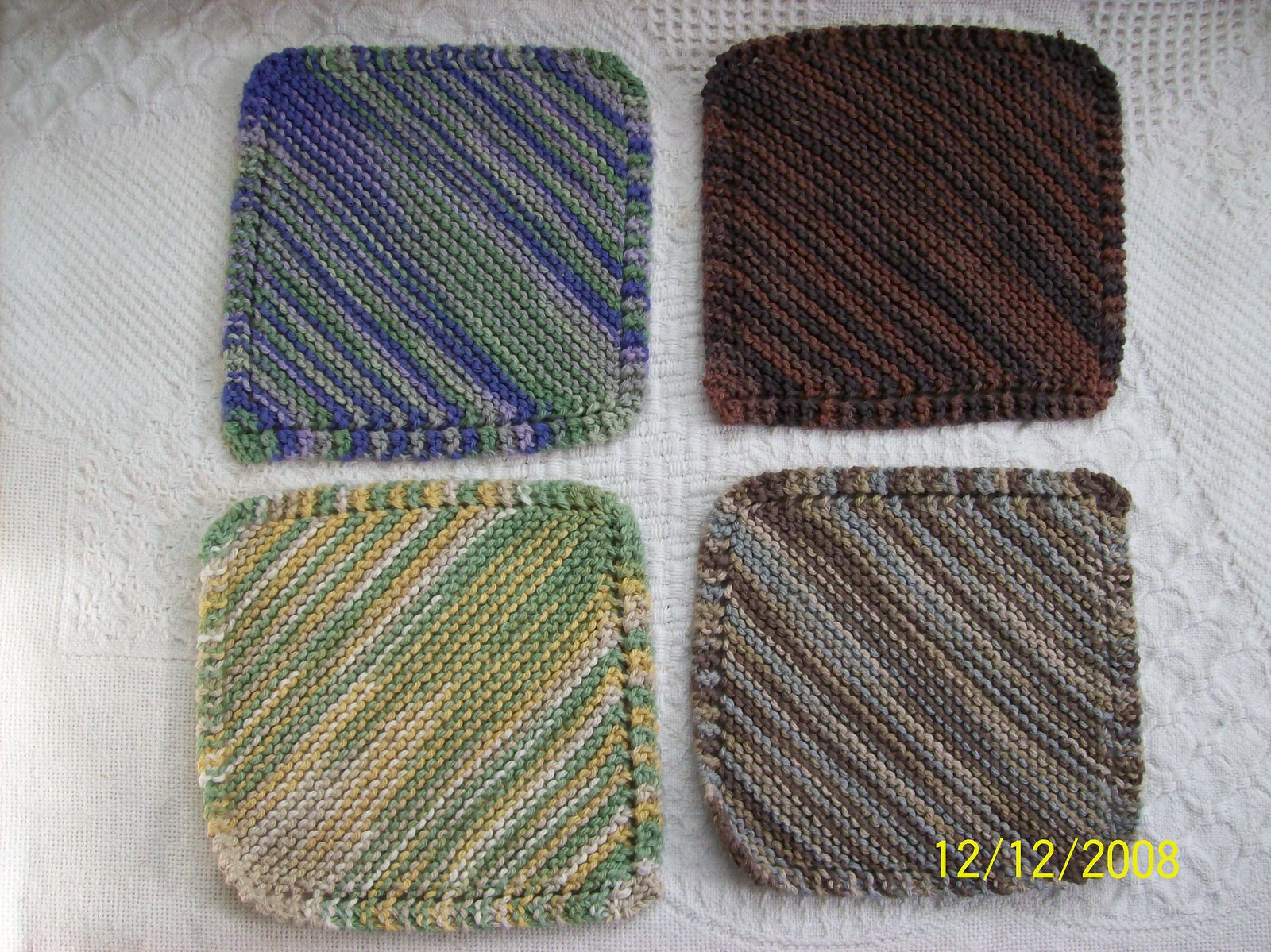This is a detailed photograph featuring four square-shaped cloth coasters, neatly arranged in a two-by-two grid. Each coaster possesses a distinct color pattern with diagonal stripes. The top left coaster showcases a blend of blue, green, and grey stripes. To its right, the top right coaster displays varying shades of brown with diagonal stripes. The bottom left coaster is adorned with stripes of green, yellow, and a greyish or beige color. The bottom right coaster features a combination of grey, blue, and brown stripes. Notably, in the bottom right-hand corner of the image, there's a yellow text date stamp that reads "12-12-2008," indicating that the photo was taken on December 12, 2008. The background of the image is set against a white fancy cloth with subtle designs, adding an elegant touch to the overall presentation.